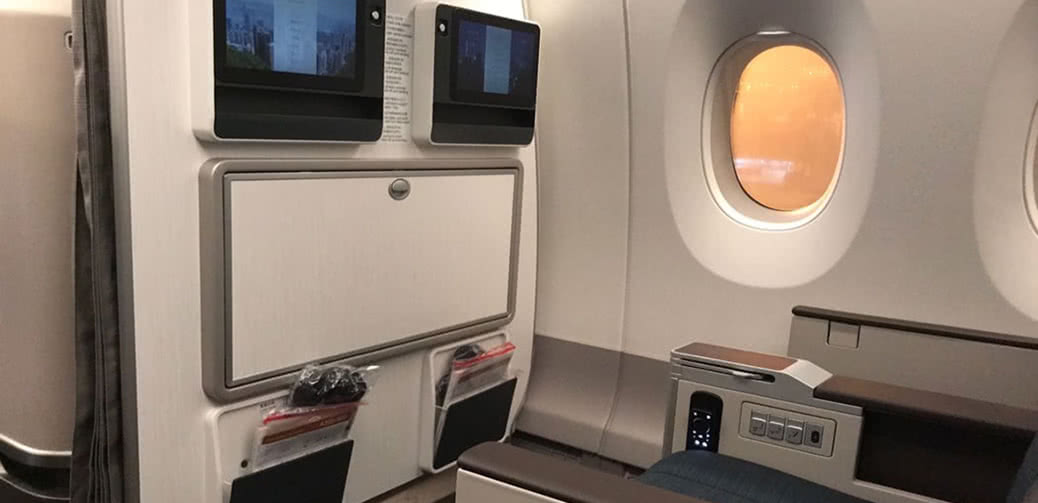This color photograph, captured in landscape orientation, presents a detailed view of an airplane's interior wall. Dominating the right quadrant, a single window occupies the scene with its shade drawn, reflecting the orange-yellow glow from an overhead light. To the left, the back of the adjacent seat features an upright, undeployed tray table. Mounted above the tray, two personal screens are visible, likely purposed for in-flight entertainment. Beneath them, dual seatback pockets bulge with magazines, safety instruction cards, and possibly oxygen masks. The airplane's wall and seat colors blend pale beige and gray tones, contributing to a sophisticated yet subdued ambiance. At the bottom right corner, the photograph captures the seat's control buttons, adjacent to the dark gray cushion peeking out from a flat section of the seat. A gray curtain subtly unfurls behind the entertainment panel on the left, adding a layer of texture to the composition. The photograph's sharp lines and meticulous details make it an attractive and visually engaging depiction of the airplane's interior.